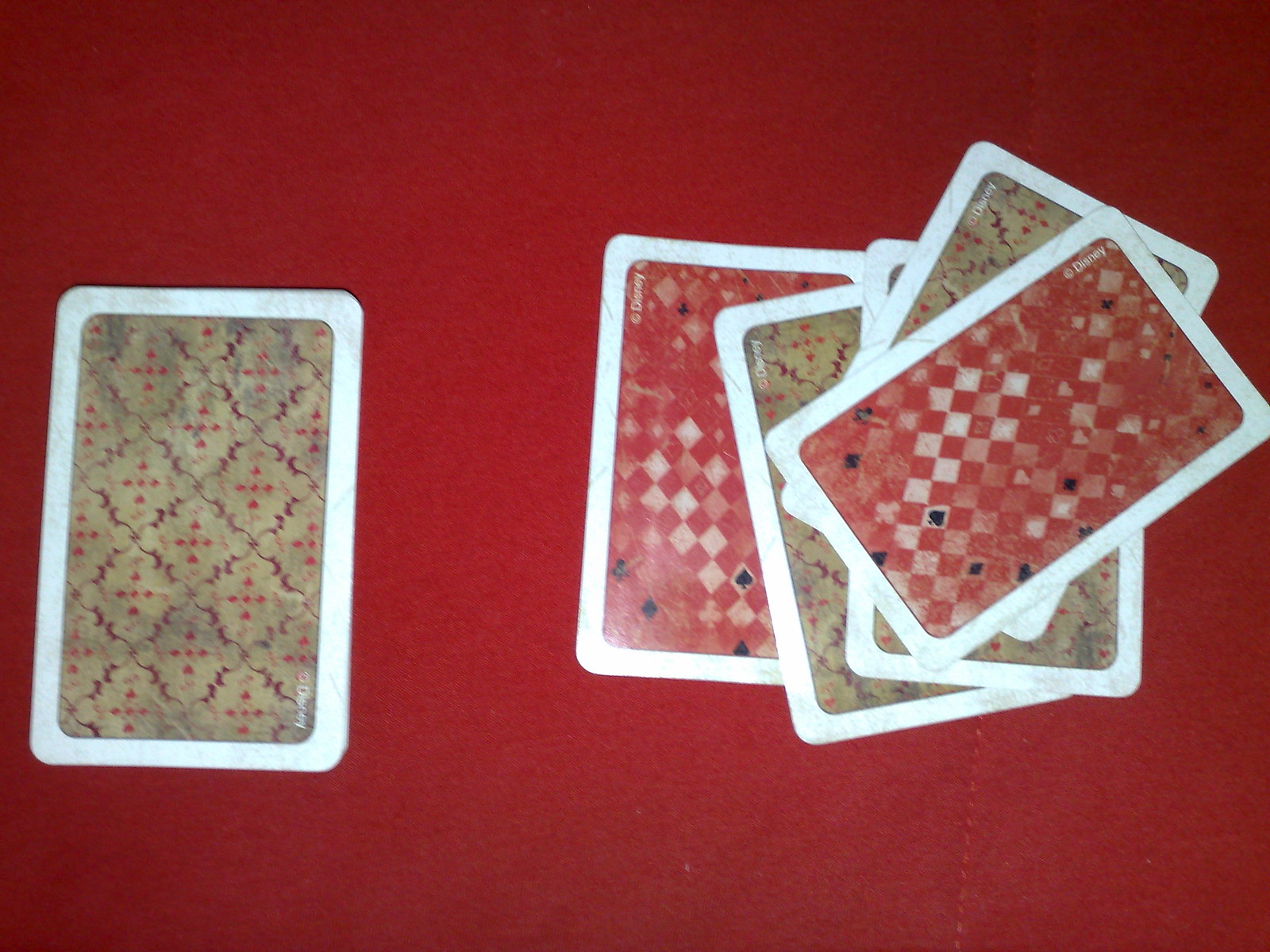A set of playing cards is displayed on a nearly featureless red cloth surface, distinguished only by a subtle sewn seam running vertically from the bottom to the top, though this seam is more prominent at the bottom. The cards are laid face down, revealing two distinct back designs, suggesting they come from different decks.

Four of the cards feature an olive green back adorned with a delicate black lace pattern forming a crisscross design. Within each crisscross opening, five red dots are arranged in a cross shape. 

The remaining two cards have a predominantly red back decorated with a checkerboard pattern in various shades of red and white. Embedded within some of the diamond shapes of this checkerboard pattern are black symbols of card suits, including spades, diamonds, and hearts, all uniformly colored in black rather than their traditional colors. 

In the upper left-hand corner of each red-backed card, there is some text that appears to be a copyright notice, beginning with a capital "D" and ending with a "Y," possibly indicating "Disney," although the exact text is hard to discern.